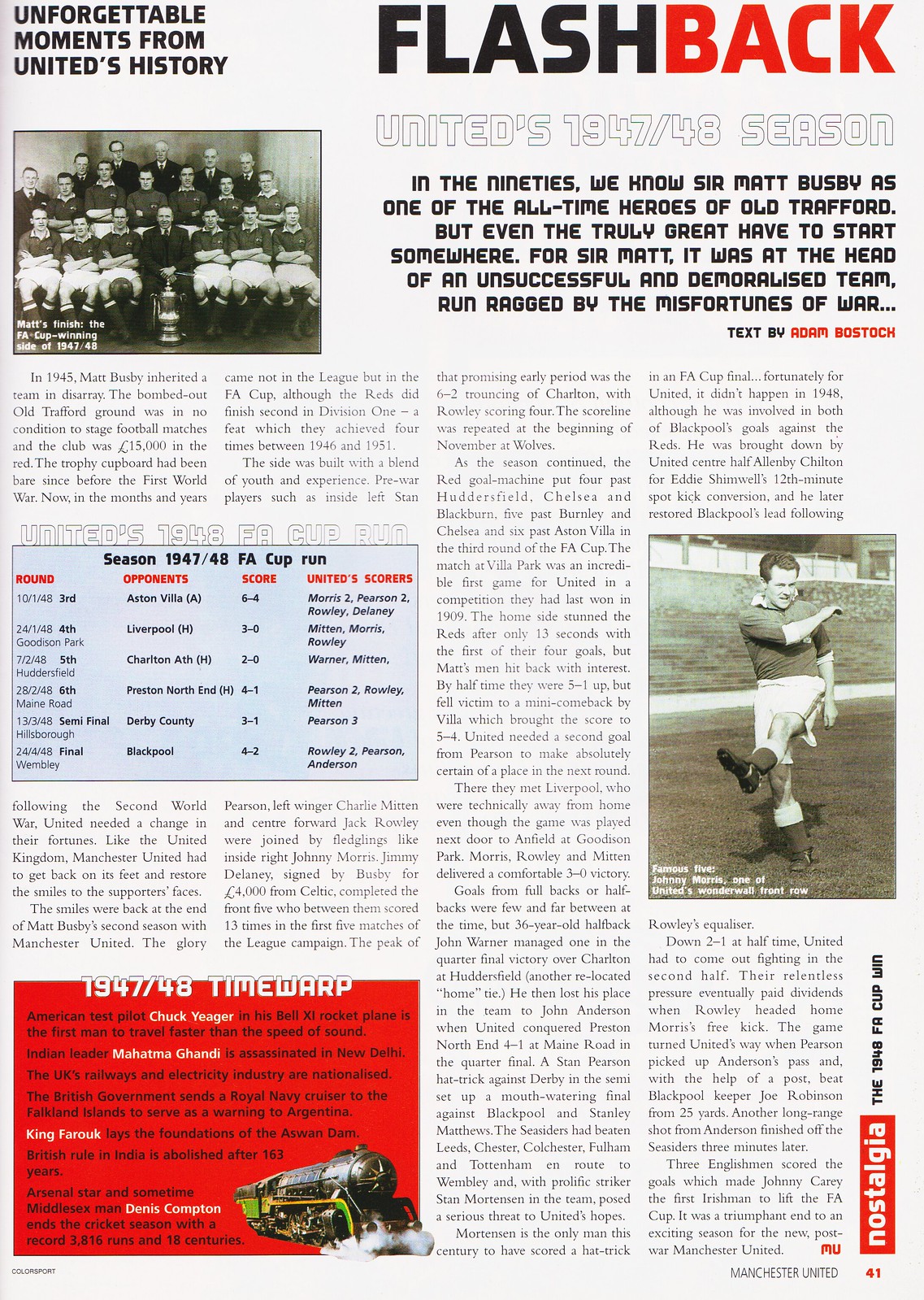This image is of a page (page 41) from a Manchester United magazine, dedicated to historical reflections on the team's notable moments. The top left of the page prominently features the title "Unforgettable Moments from United's History." The top right corner is marked with the headline "Flashback" in dual colors, black ("Flash") and red ("Back"), with the subtitle "United's 1947-48 Season" in white text beneath it. The page provides an in-depth look into the era when Sir Matt Busby, renowned in the 90s as one of the all-time heroes of Old Trafford, began his journey amidst a struggling and demoralized United team ravaged by the aftermath of the war.

The main text, authored by Adam Bostock, discusses how Sir Matt took charge of an unsuccessful team, emphasizing that even legendary figures had humble beginnings. Visual elements include photographs of Manchester United players, one image featuring a group of men (some possibly wearing masks), and another highlighting Johnny Morris from the team. Additionally, the phrase "1947-48 Time Warp" appears in the bottom left corner.